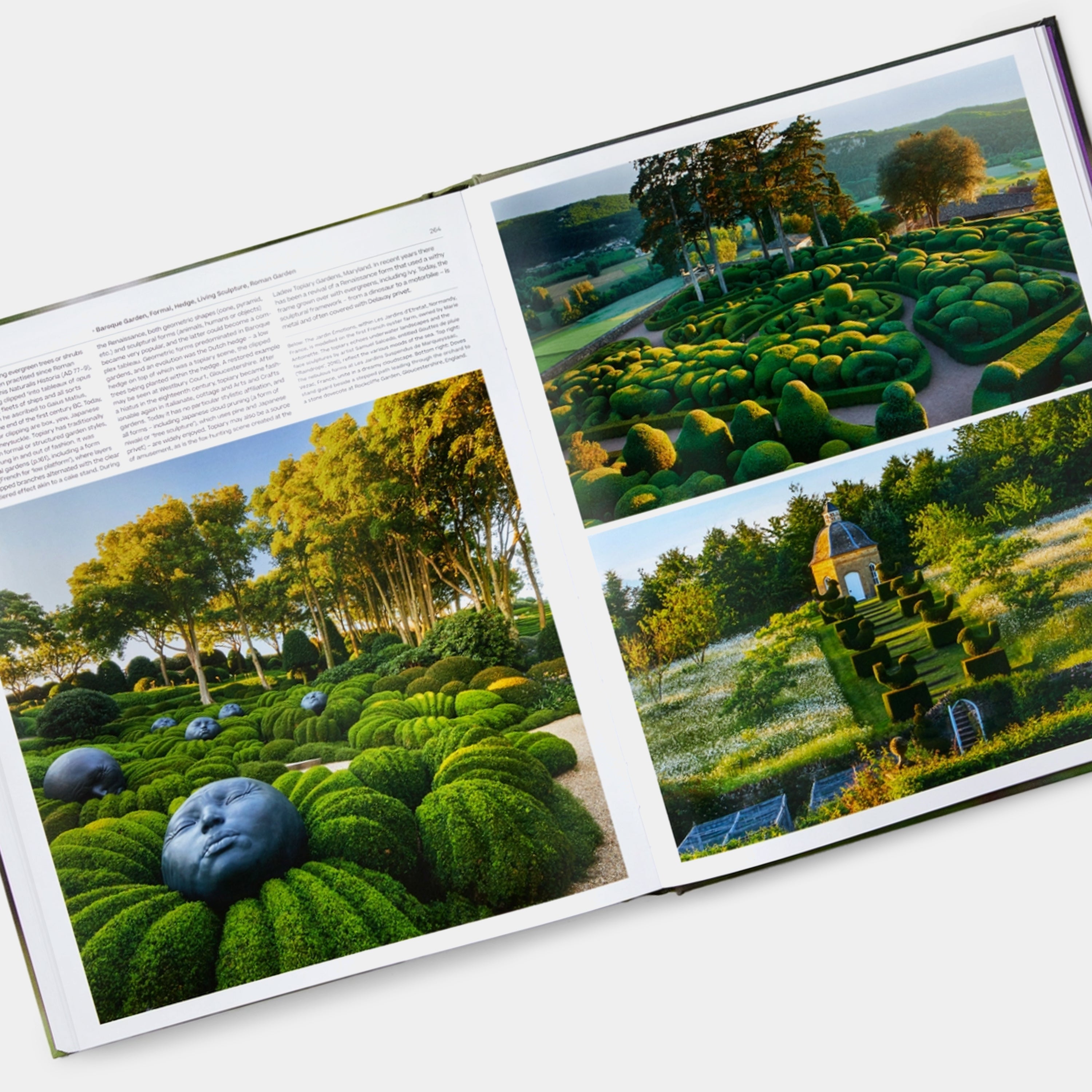The image depicts an open book on a white background. The left page features a small amount of unreadable text at the top, arranged in three columns, above a large illustration that spans the bottom two-thirds of the page. This illustration shows a garden with well-manicured bushes, each containing a central grayish-blue face with closed eyes and a frowning mouth, reminiscent of digitized or AI-generated art. 

The right page of the book displays two smaller images stacked vertically, each occupying half the page. Both images also depict garden scenes. The top image showcases curvy walking paths winding through a well-manicured garden, resembling a garden maze. The bottom image, set at the base of the right page, features a small pagoda or gazebo situated on a hill, with steps leading up to it, flanked by neatly trimmed bushes and greenery. The overall aesthetic has a video game or digitized feeling.